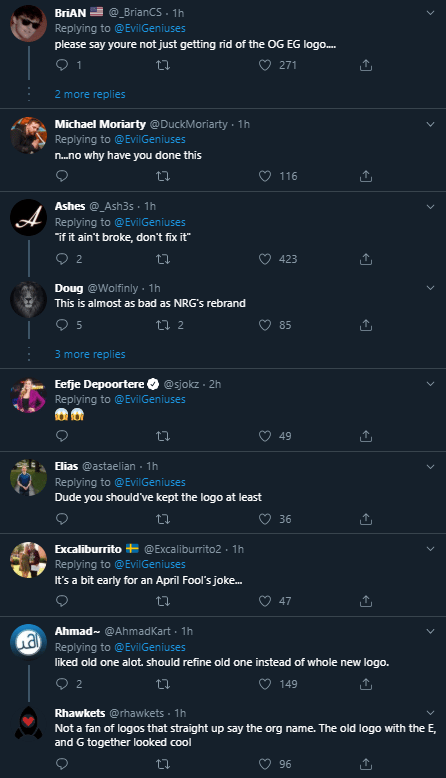Here is a cleaned-up and detailed caption for the image:

---

A lengthy, rectangular screenshot of a Twitter comment section, showcasing multiple replies to an original tweet that has been cropped out. The background is black, indicating that the app or phone is set to night mode. At the top of the screenshot, a user named Brian, whose username is displayed in white along with a flag emoji, has the handle @BrianCS. His reply, posted one hour ago, is directed at @evilgeniuses and reads, "please say you're not just getting rid of the OGEG logo." This tweet has garnered 271 likes and one comment. Below Brian's tweet are nine other replies. Each tweet in the screenshot features icons for a chat bubble, retweeting, liking, and sharing at the bottom of the respective replies.

---